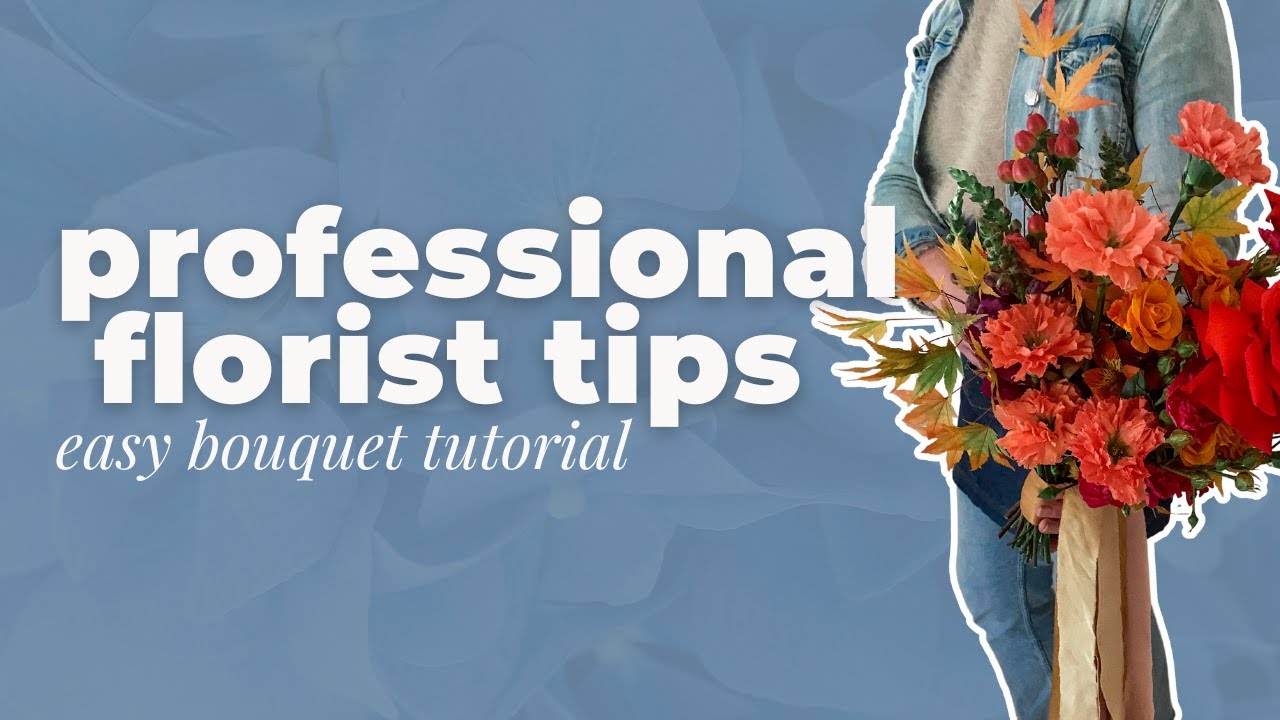The poster features a bluish-gray background with prominent, white lowercase block lettering reading "professional florist tips" and underneath, "easy bouquet tutorial." Positioned on the right side of the poster is the silhouette of a person visible from the shoulders to the ankles. The person is wearing a denim jacket with silver buttons, a gray shirt, and blue jeans. They are holding a large, colorful bouquet of flowers, wrapped in craft paper and tied with a big yellow ribbon. The bouquet, which takes up most of their body, showcases a variety of open flowers including yellow, pink, orange, and red blooms, with some greenery and brown leaves interspersed. Among the flowers, there are carnations, lilies, daisy-shaped flowers, roses, and what look like peonies and eucalyptus, all complemented by the fall-themed maple leaves. The person is holding the bouquet by its stems, near the ribbon.